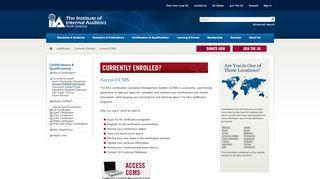This image captures a miniature screenshot of a website. Despite attempts to zoom in for readability, the top navigation bar can be seen spanning the full width of the screen with a gradient from darker blue at the top to a lighter shade at the bottom. The left part of the bar is blank, but just past the center toward the right, it contains a horizontal menu consisting of six items labeled numerically from 1 to 6. Directly beneath this bar, a lighter blue section is present, featuring the website's name and a logo that appears to include the letters 'I' and 'A'. Further down, another horizontal menu in a lighter blue hue is visible. Prominently displayed in the main central section of the website is a red bar with the text "currently enrolled."